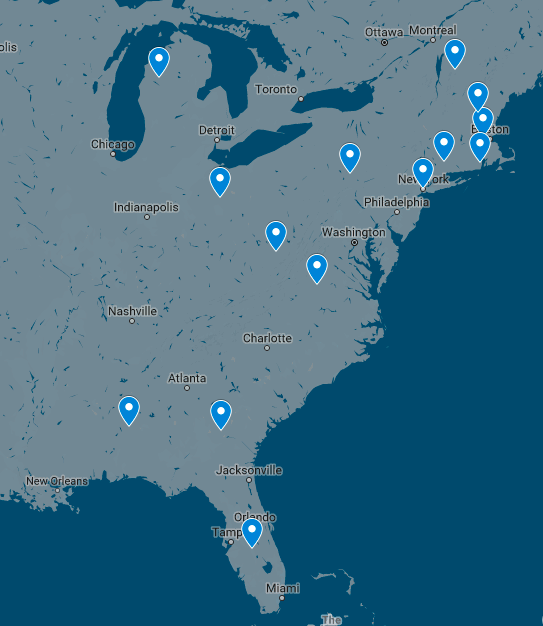This detailed map highlights the eastern regions of both the United States and Canada, extending to the central parts of the U.S. and lower regions of Canada. The land areas on the map are depicted in a gray color, while the water bodies, including the oceans and the Great Lakes, are illustrated in a dark blue. Numerous blue pins are scattered across the map, though their specific significance is not indicated.

Several major cities are prominently marked and labeled. In the United States, these cities include Miami, Tampa, Orlando, Jacksonville, New Orleans, Atlanta, Charlotte, Nashville, Indianapolis, Chicago, Detroit, Washington, Philadelphia, Newark, and Boston. In Canada, the cities of Montreal, Ottawa, and Toronto are also labeled. The map provides a clear, visual representation of these urban centers along with their geographical placement within the described regions.